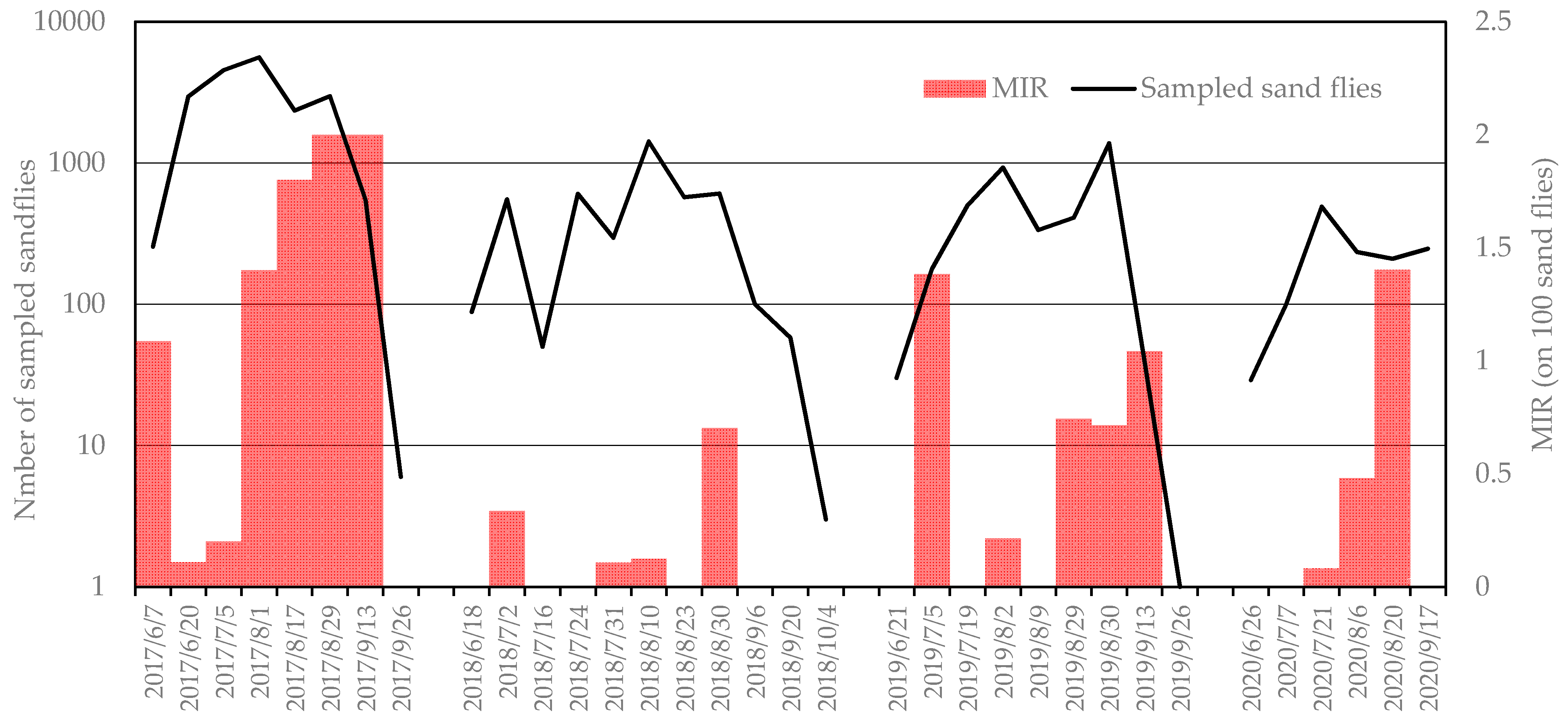This photograph features a detailed chart with a white background, prominently displaying data using pinkish-red bars and thinner black lines. On the left side, the chart is labeled "Number of Sampled Sandflies," while the right side indicates "MIR on 100 Sandflies." The horizontal axis at the bottom spans dates from June 7th, 2017, to September 17th, 2020. The pinkish-red bars represent the MIR values, and the black lines depict the number of sampled sandflies. Red bars appear throughout the chart but are absent on several dates, whereas the black lines are more consistently present, though not continuous. The overall color scheme includes cream, magenta red, or salmon red, with black text and lines, providing a clear visual distinction between the MIR and sampled sandfly data across the timeline.